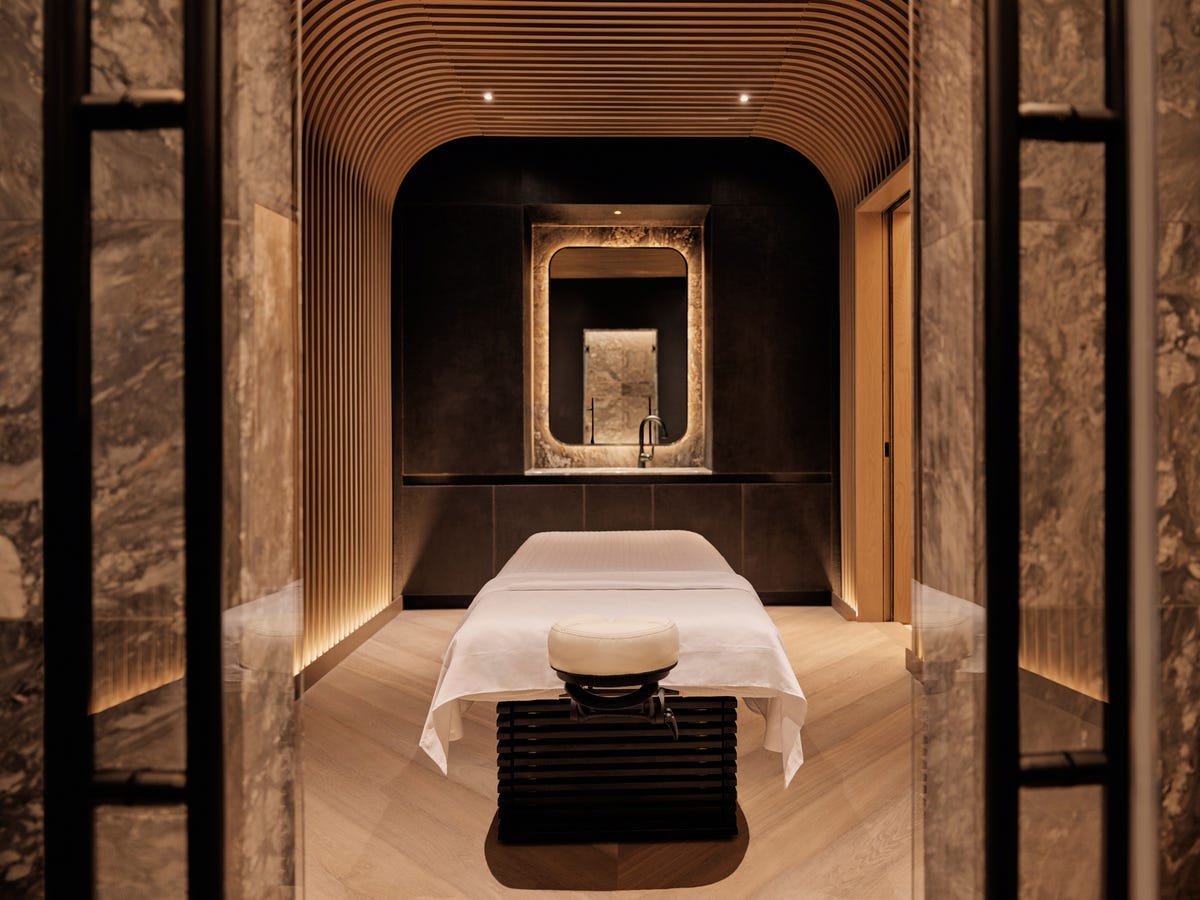The image depicts a minimalist room featuring a bed centrally positioned and draped with a pristine white cloth. The room boasts sleek white flooring and a ceiling adorned with geometric lines that extend to the walls. To the left, there is a semi-transparent doorway that offers a glimpse into an adjacent space. A round pillow lies at the forefront of the bed.

On the back wall, which contrasts the rest of the room with its rich dark brown hue, there is an elegant mirror framed in brass, adding a touch of sophistication. Below the mirror, subtle lighting fixtures provide a soft, ambient glow along the lower part of the wall. The ceiling is equipped with two additional lights, ensuring the room is well-illuminated.

To the right of the mirror, there is a sink and a doorway that might either be an entrance to another room or an elevator—it’s unclear. The bed rests atop a ribbed, rubber-like base, reminiscent of the boot of a shock absorber, enhancing the room's modern and industrial design elements.